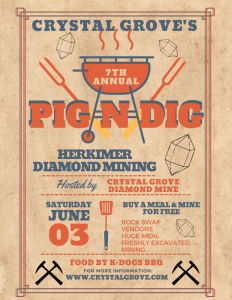The poster is an advertisement for the 7th Annual Crystal Grove's Pig and Dig event, celebrating Herkimer diamond mining. Set against a beige background with various orange and blue designs, the poster prominently features bold orange lettering for "Pig and Dig" and "June 3rd," accompanied by an orange spatula. The event details include "Saturday, June 3rd" and emphasize that attendees can "Buy a Meal and Mine for Free." Decorative elements such as sketches of diamonds and orange forks embellish the poster, conveying the mining theme. There is a drawing of a grill with a blue trim and additional details like "Rock Swap Vendors," "Huge Meal," and "Freshly Excavated Manning." The event features food by K-Dogs BBQ, and more information is available at www.crystalgrove.com. The event is hosted by Crystal Grove Diamond Mine.